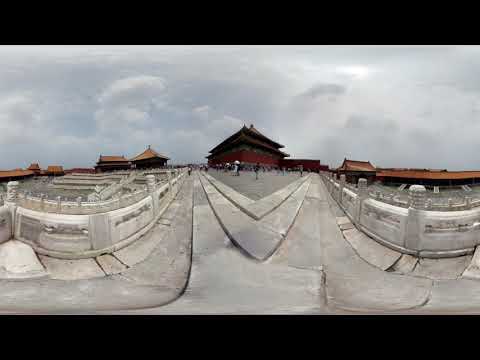This photograph, taken with a fisheye lens, captures a bustling town center with Asian architectural elements, suggesting a location in China or Japan. Dominated by a gray, cloud-filled sky, the scene feels both laid-back and touristy. In the center, a prominent reddish-brown building with traditional sloping, triangular rooftops stands out, resembling a Chinese temple. The red color, important in Chinese culture, along with the distinctive architectural style, supports this identification. Surrounding the main structure, other buildings with orange or red roofs can be seen, contrasting against the long concrete walkways and whitish-gray concrete walls that frame the area. The entire scene is set against a backdrop of hazy mountains, creating a muted yet intriguing atmosphere. Visitors and tourists are visible along the pathways, adding life to this dreary yet culturally rich setting.